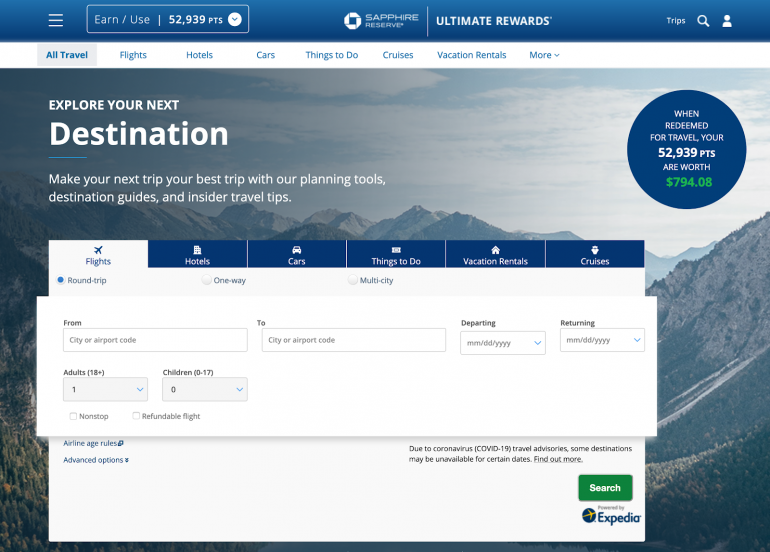**Detailed Caption:**

At the top of the image, there is a sleek header that appears almost three-dimensional. The header features a gradient of dark blue hues, with the edges being a deep blue and slightly lighter towards the center. On the left side of this header, three vertical white lines are displayed, indicating a drop-down menu option.

To the right of the drop-down menu icon, there is a transparent rectangular icon blending seamlessly into the blue background. This icon has a white border and contains light white text that reads "earn/use". Adjacent to it, a brighter white vertical divider separates this section from a bold white text displaying "52,939" in large numbers, with smaller white lettering underneath stating "PTS" all in capital letters.

Towards the right edge of the header, there is a circular white icon containing a blue downward-pointing arrowhead. Further right, a distinctive sapphire icon, resembling an octagon with four thick white borders, is present. Next to this icon, the word "SAPPHIRE" is written in bold, capital white letters.

Beneath this, a white line acts as another divider, followed by the bold, capitalized text "ULTIMATE REWARDS", accompanied by a registered trademark or trademark symbol in the top right corner.

Moving down towards the center of the page, the background transitions into a picturesque mountainous region under a partly cloudy sky. On the left, bold capital white letters spell out "EXPLORE YOUR," followed by the text "Destination" with only the "D" capitalized and larger. Beneath the "D" and "E" of "Destination," a thin blue line extends slightly rightwards. In smaller white text below this line, it reads: "Make your next trip your best trip with our planning tools, destination guides, and insider travel tips."